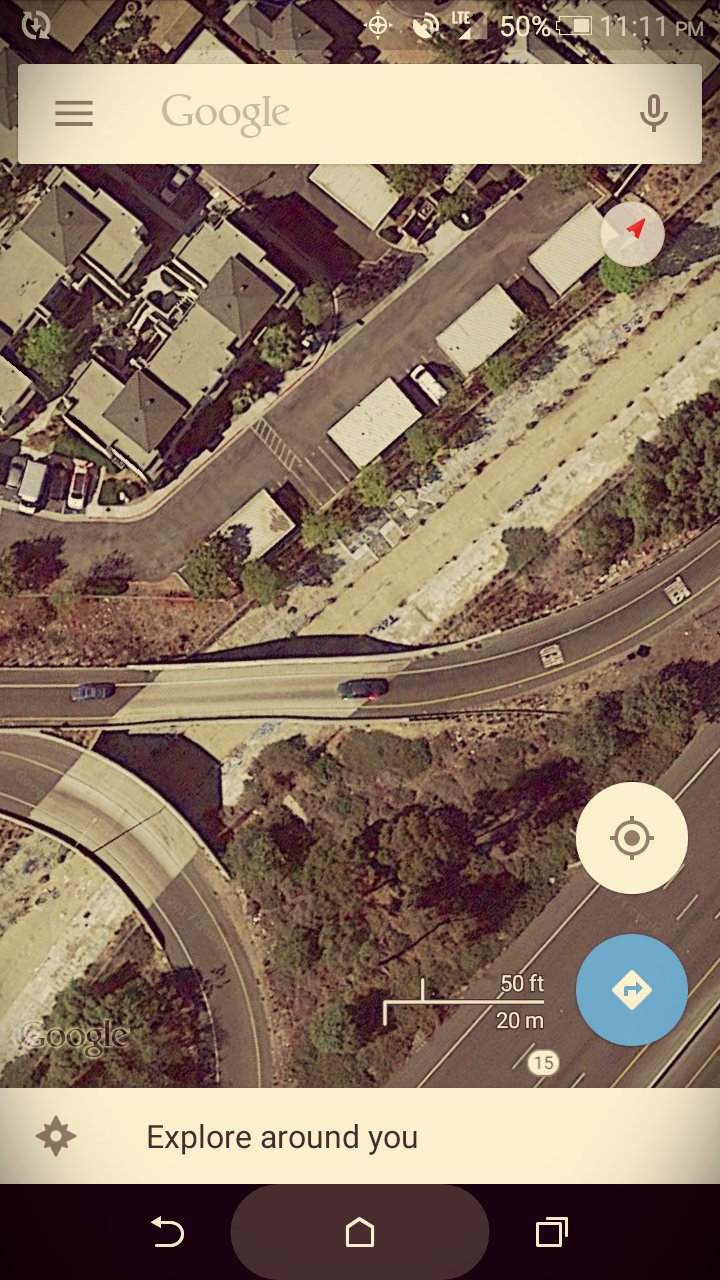**Caption:**

This sepia-toned image, taken from a cell phone or tablet, showcases an overhead view from Google Maps. The scene is dominated by three distinct roadways, with the upper section appearing densely populated. Every element in the image, including the Google search bar, is rendered in shades of tan and brown, contributing to the nostalgic sepia aesthetic.

At the very top of the image, the Google search bar is visible featuring the Google microphone icon on the right side, and the word "Google" displayed in sepia on a tan background. In the top-right corner, familiar phone icons like LTE, battery status (50%), and the time (11:11) are present.

In the bottom right corner, navigation icons are seen: the top one is a compass on a white background, and below it, an icon with a blue arrow on a white diamond set against a blue background. In the center of the image, a white line serves as a scale legend, indicating distances of 50 feet or 20 meters.

Additionally, on the bottom left, there's the curvature of a road entering from the corner that arches over toward the bottom left. A white bar near the bottom contains the text "Explore Around You" in gray letters. Along the bottom of the screen, the navigation buttons – back arrow, home, and extra window – are visible on the right-hand side.